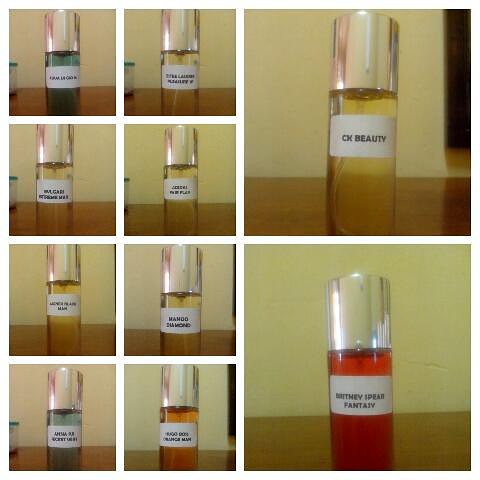The image is a compilation of ten smaller images, arranged in a grid, much like the Brady Bunch intro. Each image is a close-up of a small cylindrical bottle with a large silver screw-top, suggesting they may be sample-sized perfumes or essential oils. All the bottles are clear glass, containing various colored liquids – including clear, light blue, yellow, orange, and red. Each bottle has a white label with black text indicating different fragrances. The labels on the two larger, more prominent images read "CK Beauty" and "Britney Spears Fantasy." The smaller images, difficult to read, are organized into two rows of four on the left side. All bottles are set against a whitish background on a brown table, highlighting their simplicity and elegance.